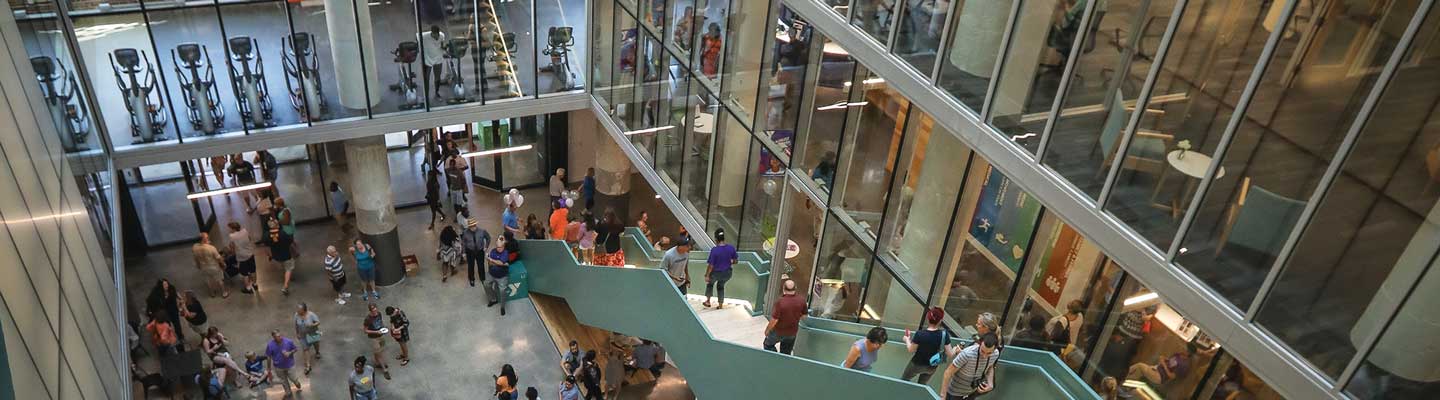The image depicts a multi-level mall from a high vantage point, likely the third floor, overlooking a bustling area filled with people. The composition is a long horizontal rectangle, which limits the depth perception of what is near or far. The focal point is a prominent green staircase with baby blue handrails and sidewalls, bustling with people moving up and down between floors. Surrounding the central area with polished concrete flooring are glass walls through which various levels of the mall are visible. On the second floor, to the left side of the image, there's a series of exercise equipment, including bikes, while the right side features lounging areas with tables and chairs. The top third floor displays stores with clothing on display and a couple of lounge chairs and a table. Lights hang above, adding to the mall's vibrant atmosphere.